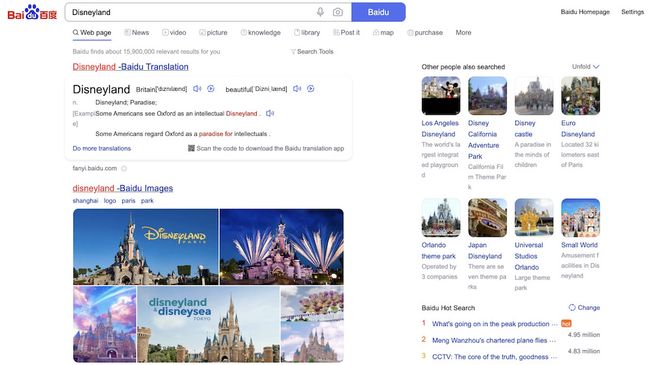This image depicts a website interface, specifically the homepage of Baidu, a popular Chinese search engine. At the top, a prominently displayed search bar contains the text "Disneyland," suggesting a recent or example search term. A blue search button adjacent to the search bar is labeled "Baidu."

Below the search bar, there is a navigation menu offering various categories for search results: Web Page, News, Video, Picture, Knowledge, Library, Post It, Map, and Purchase More. The webpage indicates it is the Indian version of Baidu, showing approximately 15,900,000 results for the search term "Disneyland," though the exact number is somewhat unclear due to poor image resolution.

Further down, the page provides translations and contextual uses of the search term. Examples include "Disneyland Bayou" and various translations and interpretations such as "Some Americans see Oxford as an intellectual Disneyland" and "Some Americans regard Oxford as a paradise for intellectuals." The page also includes a prompt to download the Baidu Translator app, accessible via a QR code. This suggests the primary function of this Baidu page is providing translation services or information related to translations.